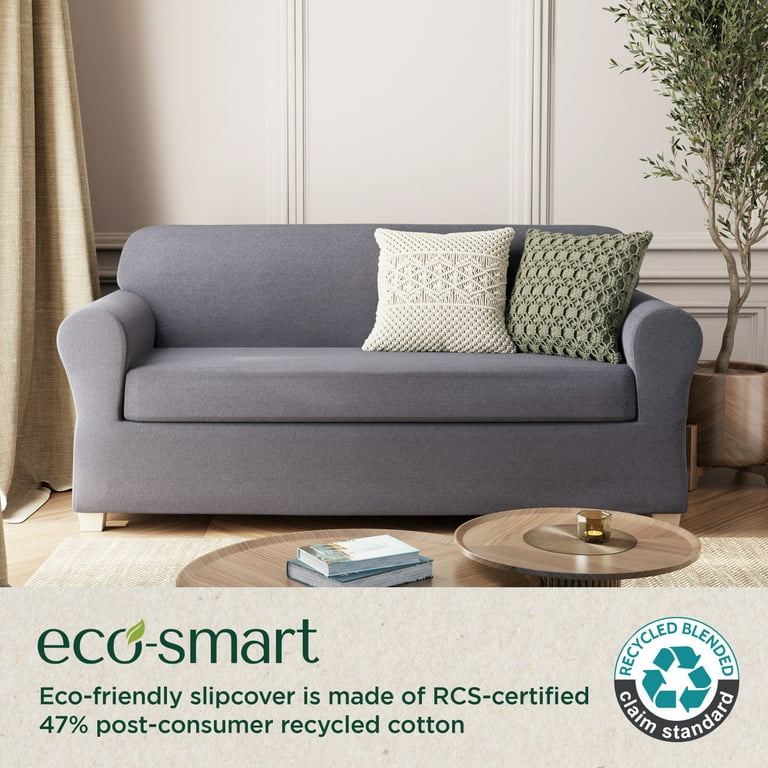This color photograph captures a cozy section of a living room featuring a centrally-placed, grayish-blue loveseat couch with rounded edges. The loveseat is adorned with two cushions: one is white with intricate embroidery, and the other is a green patterned cushion. Surrounding the couch, the room’s elements include a cream-colored wall, light wood hardwood flooring, and heavy beige linen drapes on the left. To the right of the couch, there is a potted plant with small olive-green leaves. 

In front of the loveseat, a wooden round coffee table is split into two sections, each supporting different items; one section holds two books and a candle, while the other has a glass cup. The image also features text below the scene which reads: "EcoSmart. Eco-friendly slipcover is made of RCS certified 47% post-consumer recycled cotton." To the right of the text, there is a logo with the recycling symbol and the words "Recycle Blended Claim Standard."